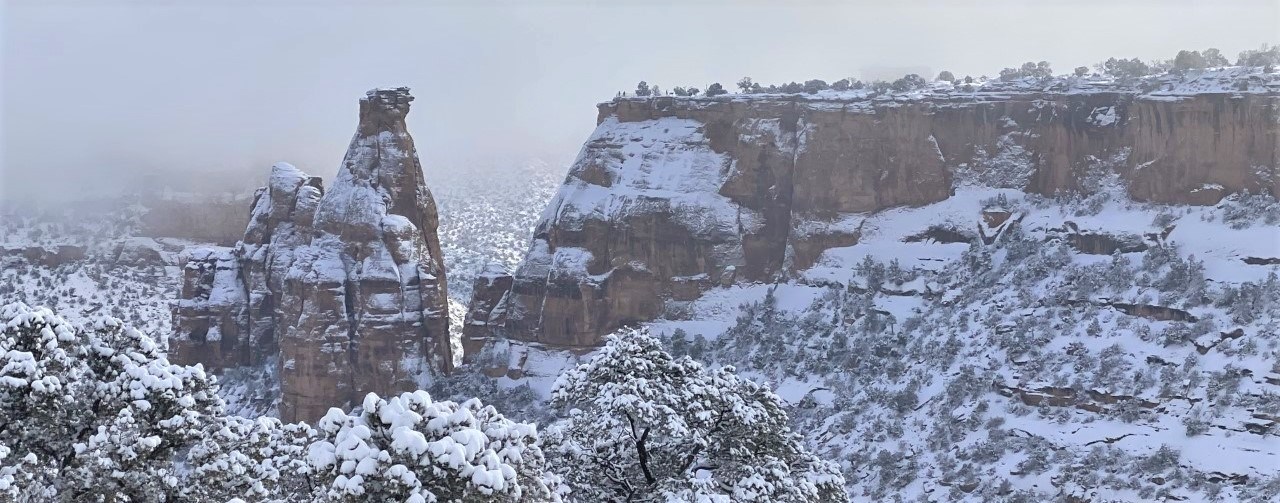This color photograph, wider than it is tall, captures a vivid winter scene in a rugged desert landscape reminiscent of the Canyonlands, possibly in regions like New Mexico, Arizona, or Colorado. Dominating the image is a snow-dusted mesa that stretches from the middle to the right edge, its flat-topped, reddish-gold surface standing in stark contrast to the white snow. The mesa is complemented by a smaller flat-topped pillar in the foreground, similarly adorned with snow. Sparse vegetation is visible, with snow-covered trees scattered throughout the landscape, particularly in the foreground. The slopes of the mesa are steep, with patches of greenery peeking through the snow. The background fades into a dense fog or haze, obscuring any further details and blending the horizon seamlessly into the sky. The overall scene is devoid of any people, structures, vehicles, or mechanical objects, emphasizing the natural, serene beauty of this snowy desert environment.